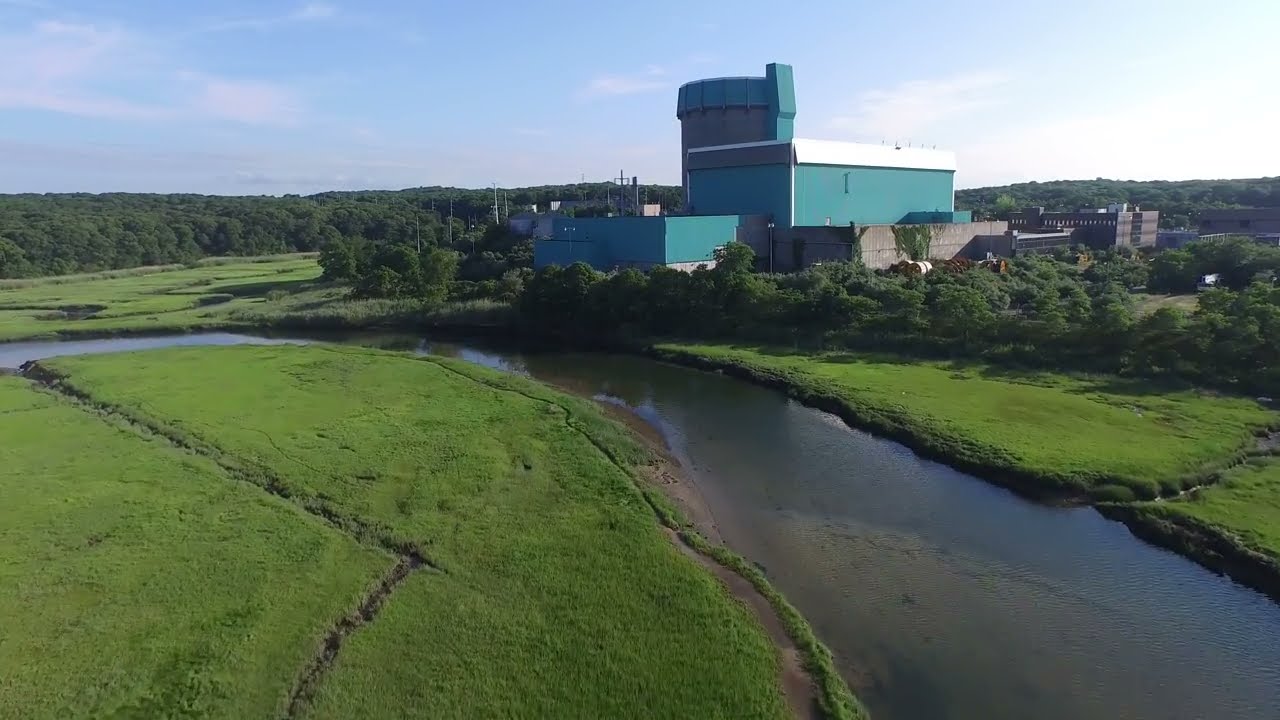The image depicts a vast, sunlit grassy field, predominantly green with various shades, set outdoors in the middle of the day. To the right side of the field, there's a paved road lined with parked cars. Adjacent to the roadway, we can see telephone poles and scattered houses. On the left side of the field, a thin, reflective, s-shaped river meanders through the landscape. In the upper portion of the image, slightly off-center to the left, stand two tall buildings, one with a gray cylindrical top. These buildings feature green roofs and gray siding. Surrounding the field, the horizon is lined with verdant trees, under a sky filled with light blue, white, gray, and turquoise hues. The scene is serene with no text visible anywhere.